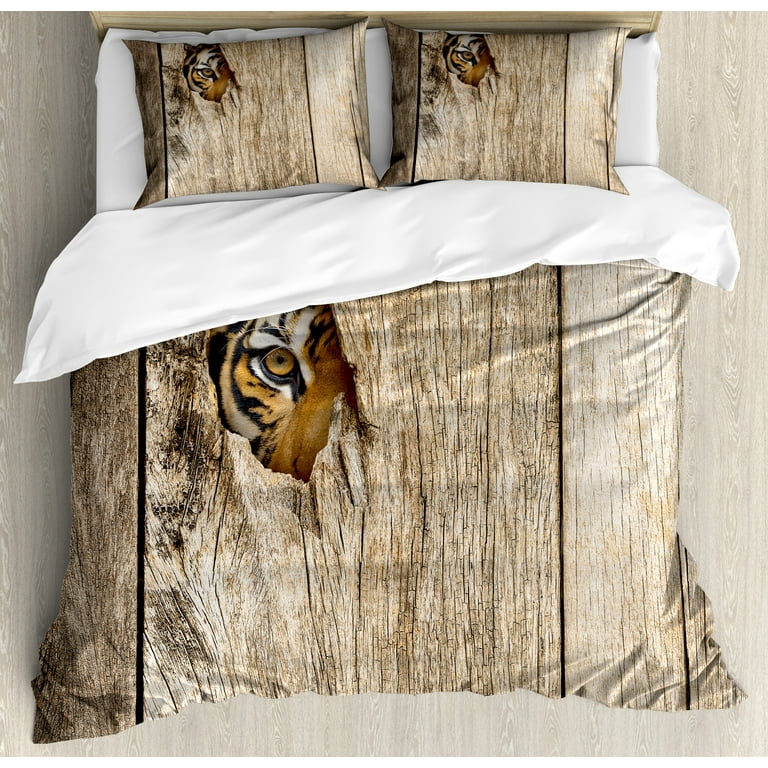This photograph captures a bed viewed from above, set against a pale, tan wood-patterned floor. The bed features two pillows, both displaying a unique design: a wood-like texture interrupted by a large knot hole through which the right eye and partial face of a tiger are visible. The darker brown hue dominates the left side of the pillow's design, while the right side is a lighter brown. The comforter mirrors this striking motif, creating a cohesive look with the pillows. Both the pillows and the comforter reveal their white undersides, while the white sheets underneath add a crisp contrast. The headboard is a subtle tan beige, complementing the overall color palette of the room.